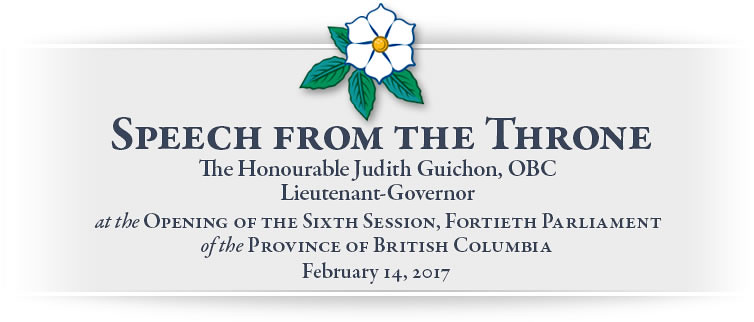The image is a formal announcement with a centered white flower featuring a vibrant yellow center, encircled by six white petals outlined in blue, and accompanied by four green leaves with a slight blue tint. The background is a subtle gradient from gray to white at the edges, providing a clean and serious tone.

At the top, the text reads "Speech from the Throne" in bold, followed by, "The Honorable Judith Guichon, OBC, Lieutenant Governor," indicating her role and honorifics. The announcement continues with, "at the opening of the Sixth Session, Fortieth Parliament of the Province of British Columbia," providing context for the event, and concludes with the specific date, "February 14, 2017." The text is centered and primarily appears in a dark gray or very rich dark green, contributing to the formal and distinguished style of the image. The overall design emphasizes the text and floral emblem, suggesting a logo-like presentation for this significant governmental event.